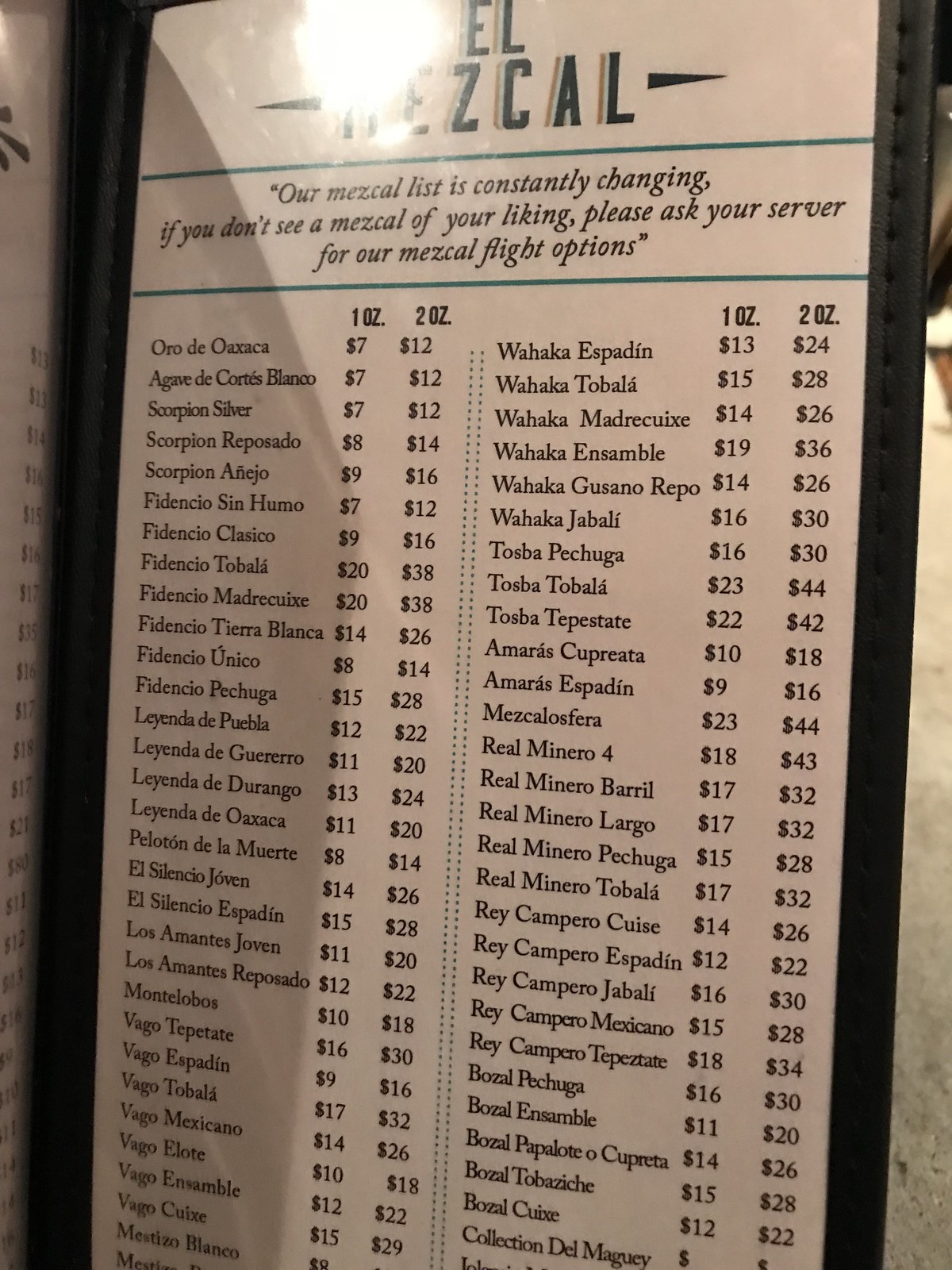This is an image of a drink menu, specifically a Mezcal list, photographed straight on and propped up vertically. The menu is encased in a black vinyl frame with plastic over it, and it's illuminated by a bright white light at the top. The light partially obscures the name of the establishment, but the visible "EL" and "Mezcal" can be seen. The menu states, "Our Mezcal list is constantly changing. If you don't see a Mezcal of your liking, please ask your server for our Mezcal flight options."

The menu features two long rows of Mezcal options, each entry detailing the type of Mezcal along with pricing for one-ounce and two-ounce portions. Although the listings appear almost alphabetical, they are out of order. In the background, on the right side of the image, there is a blurred landscape, possibly indicating a kitchen table or a shelf, but it is not clearly distinguishable.